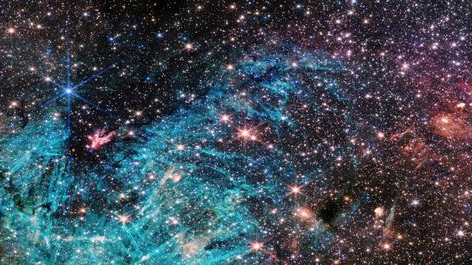The image appears to be a close-up photograph of a galaxy set against a dark, nearly black background teeming with a multitude of stars varying in size and brightness. The scene features a striking blue, gaseous nebula swirling like a wave in the center and extending to the right side of the image. The upper left corner is illuminated by a radiant blue light that could be a star, casting a glow over part of the nebula. Additionally, there are subtle pink hues scattered among the dense star field, possibly from dust clouds or starbursts, adding more depth and color variety. The stars, ranging from bright white to shades of yellow, orange, and red, twinkle against the deep, richly dark canvas of space. The intricate patterns and striations within the blue nebula evoke a sense of motion and phenomenal celestial activity, making the whole composition a mesmerizing snapshot of the cosmos.